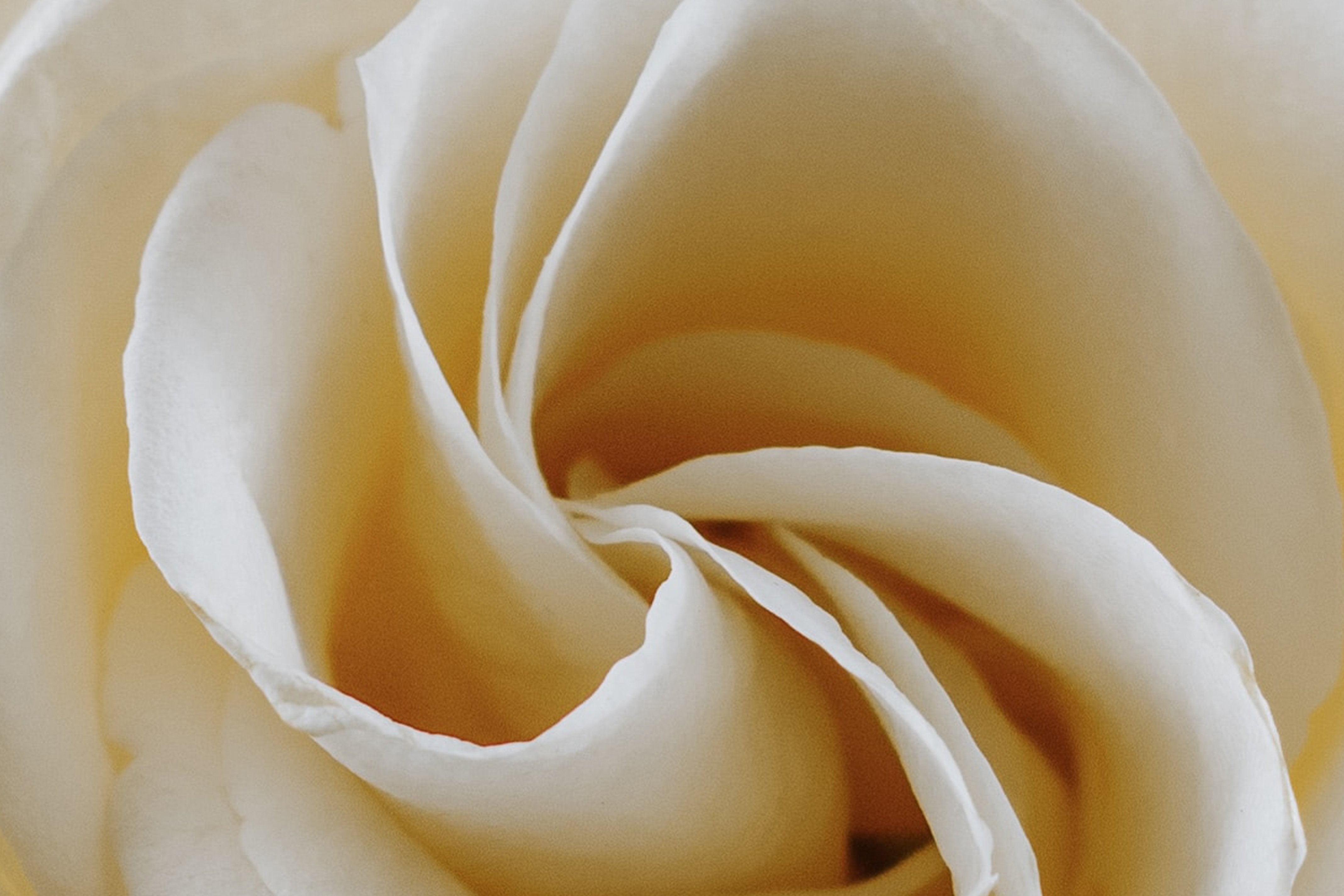This is a highly detailed macro photograph capturing the intricate center of a white rose, possibly real but with an impression of refined texture that might suggest otherwise. The entire frame is filled with the close-up of interwoven petals that gradually spiral inward, creating a mesmerizing swirl effect. The petals exhibit a gradient of colors, starting from a pure white or very light cream at the edges and blending into deeper shades of creamy beige and peach towards the center. The lighting highlights the outer rims of the petals, making them appear almost luminescent while the innermost folds are more shaded. The focus is sharpest at the core, progressively blurring towards the edges, indicating a wide aperture typical of macro photography. The photograph is horizontally oriented, showing at least eight distinct petals curling inward. Notably, the bottom right corner features a darker triangular area, providing a stark contrast against the otherwise light-dominated composition.